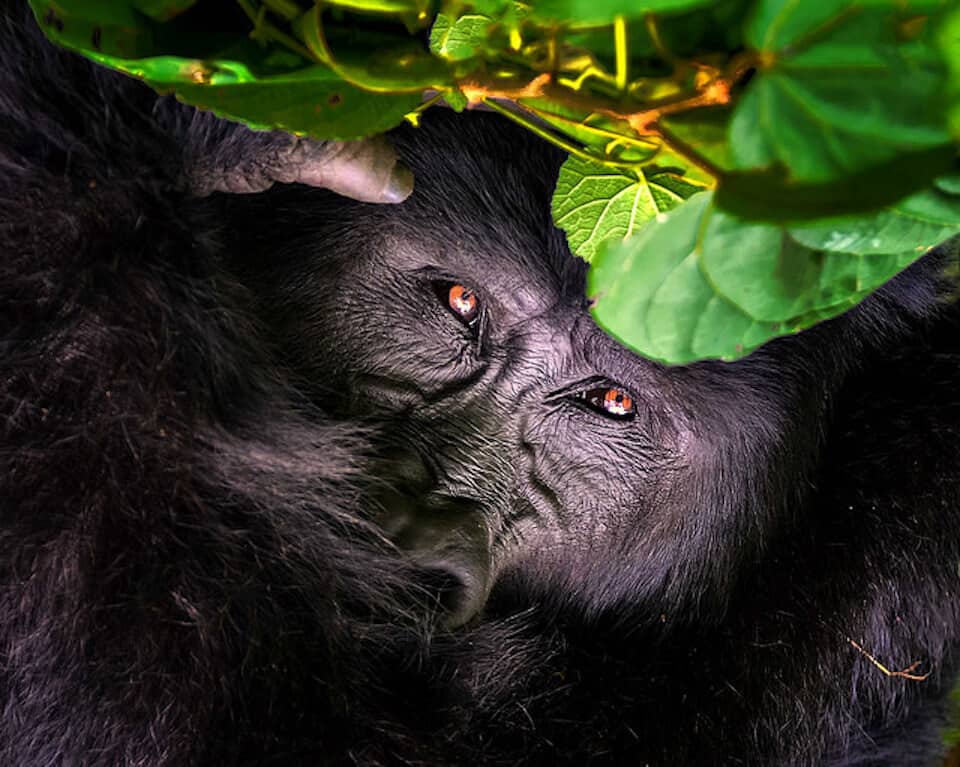In this detailed close-up image, we see a gorilla peering through green leaves, which are attached to a brown stick at the top of the picture. The gorilla's serious expression is accentuated by the wrinkles on its face, and it appears to be looking directly at us with dark, amber-colored eyes. His short, thick fur is a striking black and silverish color. The gorilla's nose and the top of its thumb are visible, suggesting that it might be using its hand to part the leaves for a better view. The overall lack of text in the image emphasizes the intense and direct gaze of the gorilla, making the photograph feel intimate and captivating.